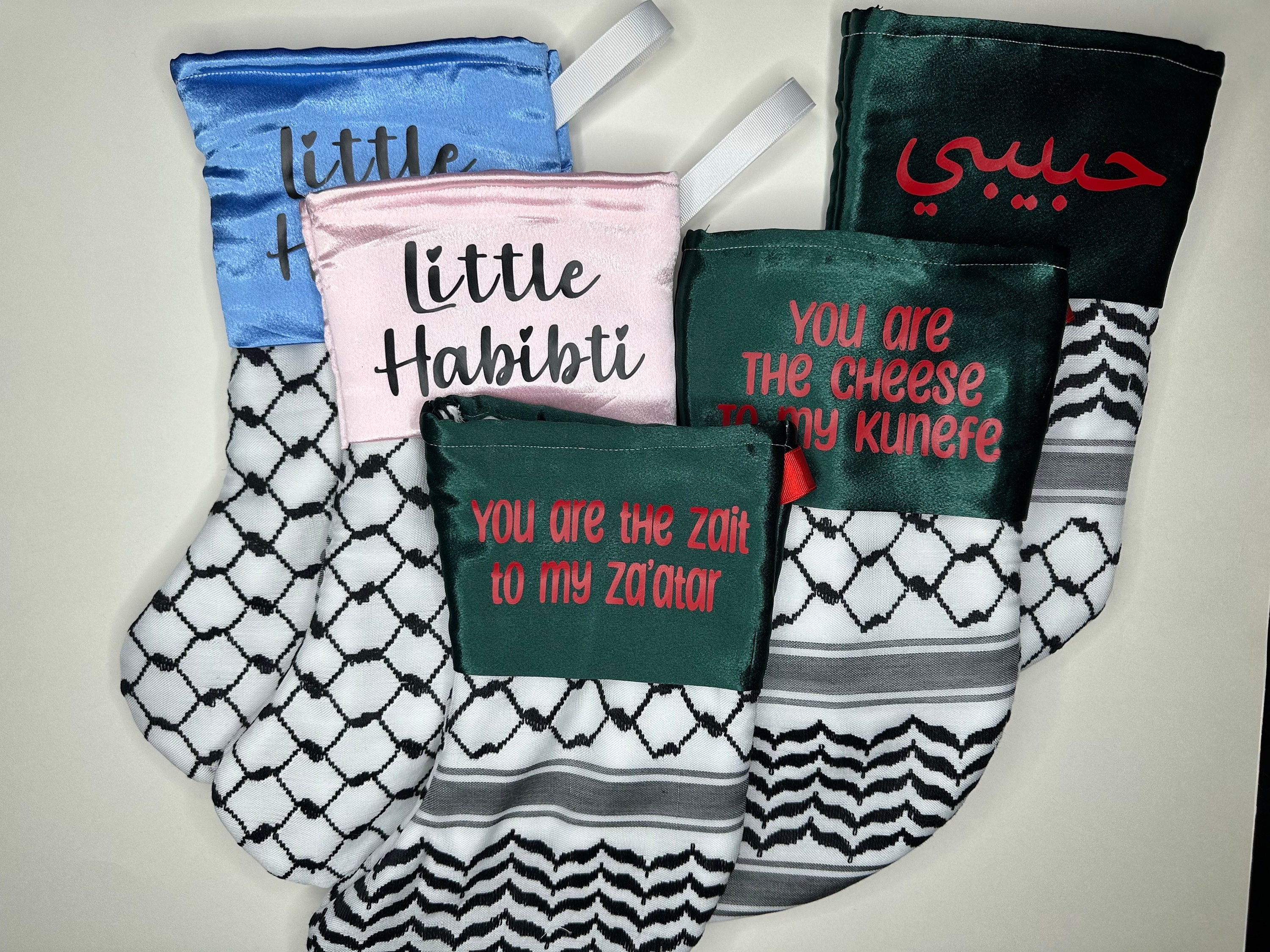The photographic image showcases a series of five stockings hanging on a plain white wall, likely indoors. The stockings feature a consistent design with the foot parts adorned in white fabric and intricate black geometric and web-like patterns, emphasized by interlocking and wavy lines along with little gray dividers. Each stocking has a distinct colored cuff with inscriptions in red text. 

Three of the stockings have green cuffs. The first green-cuffed stocking reads, "You are the Zait to my Zaatar" (Z-A-I-T to Z-A apostrophe A-T-A-R). The second green-cuffed stocking displays the text, "You are the cheese to my Kunefe" (K-U-N-E-F-E). The third green-cuffed stocking features a message in Arabic. 

Accompanying these, a pink-cuffed stocking bears the phrase, "Little Habibti" (H-A-B-I-B-T-I). The final stocking, which has a metallic blue cuff partially obscured by the pink one, also says "Little..." but the rest of the inscription is hidden. All stockings are neatly stacked vertically, contributing to a visually cohesive display.